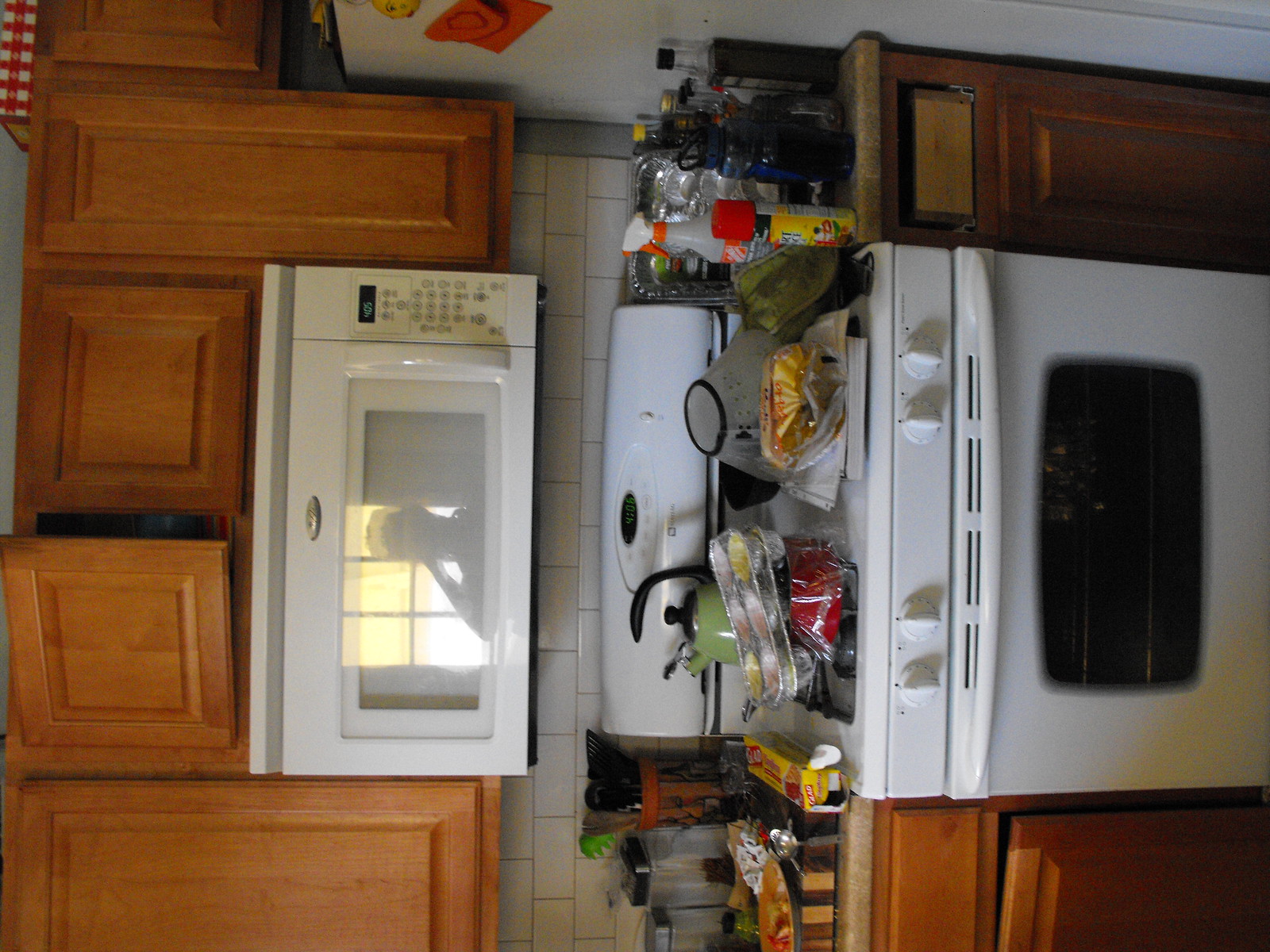The image depicts a cluttered kitchen scene where the focal point is a white stove, which is turned sideways, making it initially difficult to recognize. The stove, posing a potential fire hazard, is covered with various items including a couple of muffin pans, a green tea kettle, and a glass lamp cover. Adding to the clutter, there are additional kitchenware items like another muffin tin, as well as condiments which might include Tabasco sauce, all scattered around. To the side of the stove, cleaning supplies are visible, along with a container that possibly holds scissors. The stove area is framed by wooden paneling below, and the countertop adjacent to it is a brownish color highlighted with a striped wood cutting board. 

Above the stove, there is a microwave, also white, that appears relatively modern, although not brand new. Surrounding the stove and countertop are numerous containers, likely holding items such as spaghetti and possibly a roll of Saran Wrap or another type of plastic wrap. This entire area is cluttered with various kitchen essentials, creating a very busy and crowded appearance. One of the cabinets to the left of the stove is slightly ajar, suggesting frequent use in this heavily occupied space.